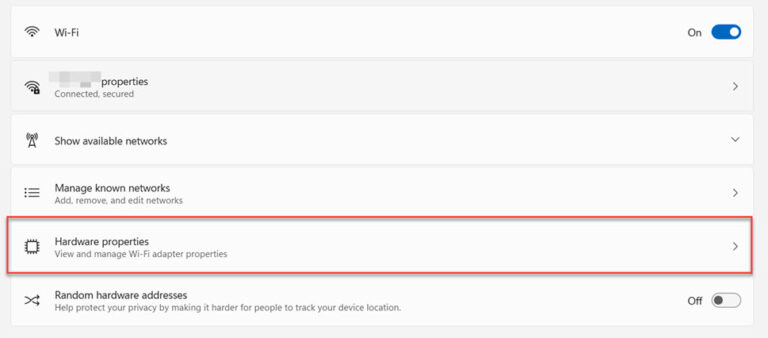The screenshot displays the Wi-Fi settings interface on a digital device, presumably a computer or tablet. The interface is bordered by a gray frame. Within this frame, six distinct areas are highlighted in white.

At the top, there is a section with a Wi-Fi icon labeled "Wi-Fi," showing the Wi-Fi state as "On." The on/off switch next to it is toggled to blue, indicating that Wi-Fi is enabled. Below this, the Wi-Fi status is displayed as "Connected, secured," implying a connection to a protected network.

Further down, there is an option labeled "Show available networks" accompanied by a drop-down arrow, allowing the user to view nearby Wi-Fi networks. The next option is "Manage known networks," which provides functionality to add, remove, or edit known networks; an actionable link suggests further modification.

A distinctly highlighted category in a red border reads "Hardware properties," which invites the user to view and manage Wi-Fi adapter properties. Lastly, there's a setting for "Random hardware addresses" aimed at enhancing privacy by making it more difficult to track the device's location; this feature's toggle switch is set to "Off."

The overall context suggests that the user might be attempting to troubleshoot a network issue, as hinted by the various detailed configuration options provided.